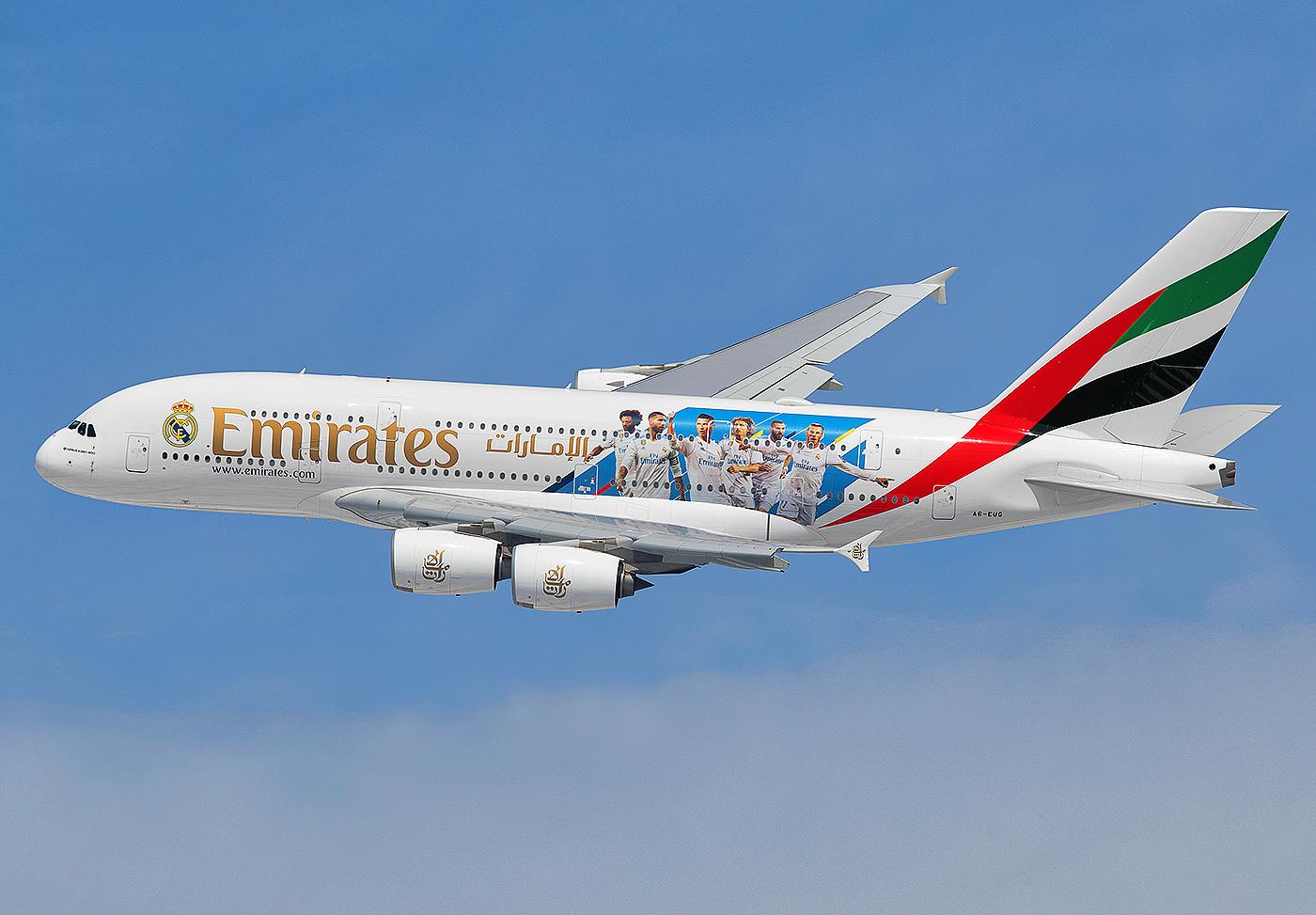In this horizontally aligned rectangular photograph, a large, white Emirates jetliner is captured in mid-flight against a vast blue sky, dotted with thin, grayish clouds below. The airliner, identified by its prominent gold "EMIRATES" print at the front, sports two distinct rows of windows and is clearly a four-engine jet, with two visible engines on its left wing and part of the right wing observable. The aircraft's tail features distinctive red, green, and black stripes. Additionally, a gold emblem follows the main branding, accompanied by some text presumed to be in Arabic. A notable image decorates the body of the plane towards the wings, depicting six men dressed in white shirts and shorts with blue lettering, appearing happy and presumably representing Emirates airline staff. The right wing displays a fascinating computer-aided design, transitioning from gray to a lighter gray at the outer section. Brigaded with the airline's web address "www.emirates.com" in gold letters, the photograph captures a high level of detail, emphasizing the grandeur and branding of the Emirates aircraft.